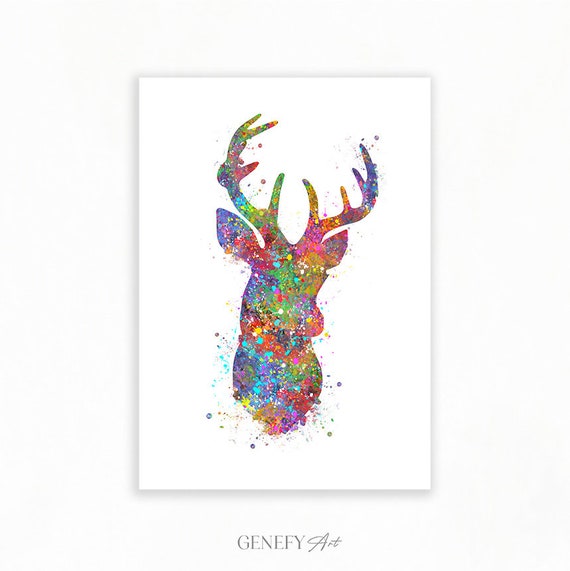The image features a striking illustration of a stag's head, reminiscent of a mounted trophy one might find on a hunter’s wall. The stag, with its prominently displayed rack of antlers, showcases roughly ten points, signifying its mature age. The artwork is rendered in a mix of vibrant, rainbow-like colors, in a style that evokes the spontaneous, abstract techniques of Jackson Pollock. The body and antlers of the deer are meticulously defined and filled with an array of hues including cyan, yellow, red, blue, purple, green, gold, and pink, creating a lively mosaic of colors that blend seamlessly into one another. Each color appears as if applied with deliberate splotches or dots of paint, lending the piece a textured and dynamic feel.

Notably, the painting does not feature the deer's eyes, with the focus instead on the vivid interplay of colors that form the animal's profile, ears, and nose. Dots and splashes of paint extend outwards from the main silhouette into the white backdrop, evoking a sense of movement and vibrancy, similar to colored snow flurries.

The artwork is set against a clean white canvas, giving it a minimalist yet striking presentation. At the bottom of the image, the piece is signed or watermarked with the name "Genify Art," where "GENIFY" is written in capital letters and "Art" in a more flowing script. The combination of meticulous detail and expressive color usage makes this painting a captivating and modern interpretation of traditional wildlife art.